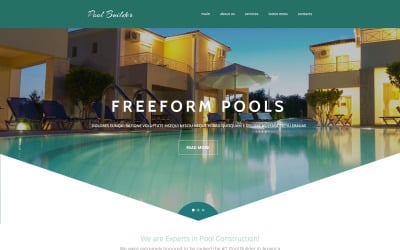This screenshot captures a low-resolution image of a website dedicated to pool services named "Pool Builder." The top section of the website features navigation tabs, though only "Home" and "About Us" are legible among the five available tabs. The header is uniquely designed, with a downward-pointing arrow shape incorporating a vibrant cyan and white color scheme accentuated by touches of yellow. The banner image showcases a luxurious pool that has a striking cyan-blue hue, set against the backdrop of an elegant, warmly-lit house.

Below the banner, there is significant white space and a bold statement that reads, "We are experts in pool construction," followed by smaller, unreadable text. The overall design suggests that the website is either under construction or incomplete. The screenshot is cropped to focus solely on the webpage, excluding any part of the browser window or desktop.